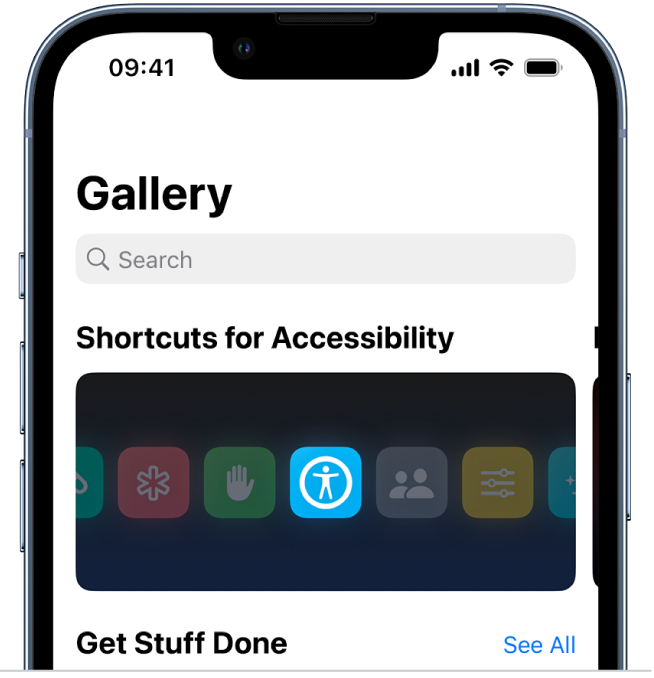The image displays the top half of an iPhone with black borders around its screen. The screen itself has a white background. In the largest font, positioned at the top left corner, is the word "Gallery." Beneath this heading is a grey search box. Further down, the text "Shortcuts for Accessibility" is visible. Below this text, there is a prominent black box featuring various coloured icons.

Among these icons, a blue one located in the center, marked by a white circle and an outlined figure, stands out prominently due to its brightness. Flanking this central icon, to its left, is a green icon with a white hand symbol and a red icon with a star. To the right of the blue icon, there is a grey icon showing the outlines of two people, and a yellow icon with a settings gear symbol.

At the bottom of this black box, the phrase "Get Stuff Done" is situated in the bottom right corner, while in the bottom left corner, "See All" is displayed in blue text.